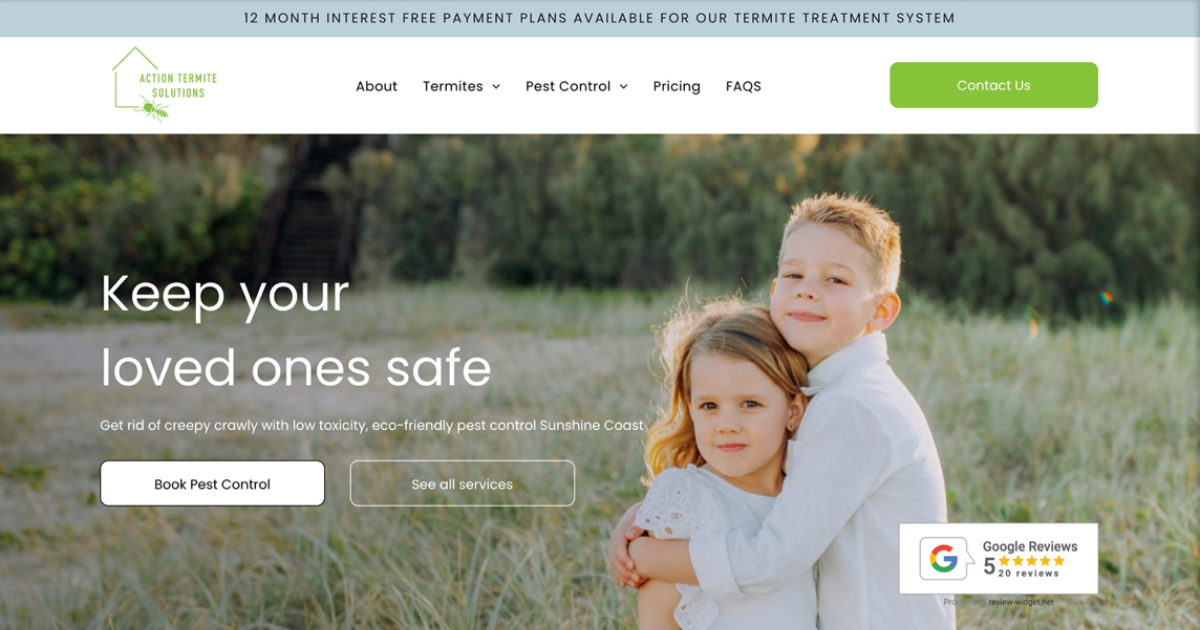Displayed on a computer screen, likely from a laptop or desktop, is a professional website for a pest control service specializing in termite treatment. 

At the very top of the page, a greyish-green strip displays a notification in black text: "12-month interest-free payment plans available for our termite treatment system."

Below this header, the website's logo—a green outline of a house with a termite icon—reads "Action Termite Solution." 

To the right of the logo, a horizontal navigation menu features options in black text: "About," "Termites" (with a drop-down menu), "Pest Control" (also with a drop-down menu), "Pricing and Facts," and a green tab labeled "Contact Us."

The main body of the screen is dominated by an inviting image set in an open field behind a house. In the foreground, a young Caucasian boy and girl with blonde hair and possibly green eyes are embracing and smiling at the camera. The boy, taller than the girl, is dressed in a long-sleeved white shirt, and the girl is wearing a short-sleeved white top or dress.

To the left of the children, text in bold white letters reads: "Keep your loved ones safe. Get rid of creepy-crawlies with low-toxicity, eco-friendly pest control Sunshine Coast." Below this, a call-to-action invites users to "Book Pest Control" or "See All Services."

The footer of the page proudly displays a Google rating of 5 stars based on 20 reviews, underscoring their commitment to quality service.